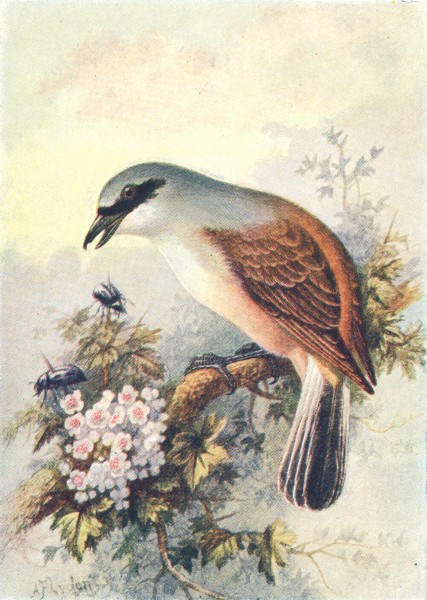In this detailed painting, the central focus is a bird perched on a rough, brown tree branch. The bird, positioned prominently in the middle, showcases intricate details: it has black legs and feet, a short, slightly curved black beak, and distinctive black markings near its eye. Its feathers display a blend of dark brown, black, and lighter tones, with the tail being notably black and white. The bird faces left, leaning slightly towards that direction.

The background of the painting is a soft, almost ethereal mix of light yellow, pink, and purple hues that evoke a serene sky with a hint of clouds. Surrounding the bird on the tree branch are vibrant elements of nature, including small green leaves and delicate white flowers with pink centers. 

There are also a couple of small black beetles visible on the lower section of the branch; one is directly below the bird's beak on a green leaf, while another is to the left. The lower left corner of the painting seems to bear a faint autograph, potentially reading "Riden" or "Flyden." The overall composition is a harmonious depiction of nature, rich in color and detail, rendered in a vertical rectangular format typical of classic art painting styles.